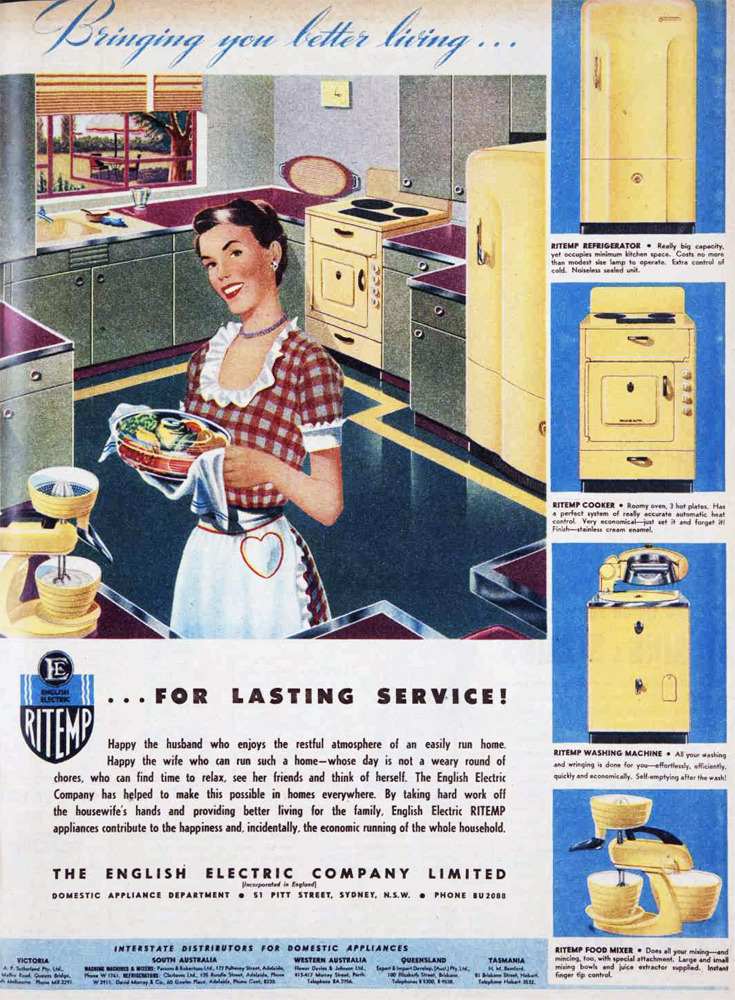This vintage print advertisement from the 1940s or 1950s, presumably a cutout from a magazine, showcases a detailed artist's rendition of kitchen appliances by the Right Temp Company, under the slogan "Bringing You Better Living." The ad features a central illustration of a cheerful woman dressed in a gingham dress and a white apron adorned with a heart on the hip and ruffles around the neckline and sleeves. She has short brown hair in a bun and holds a dish of prepared food, standing amidst her kitchen's gray cabinetry with burgundy Formica countertops. Behind her, the kitchen boasts a window with Venetian blinds, offering a glimpse into her backyard. 

On the right side of the ad, four detailed illustrations of appliances are arranged vertically on blue backgrounds: a yellow refrigerator, a yellow stove, a yellow washing machine, and a yellow stand mixer, each shown in a front view with descriptive captions. The promotional tone emphasizes the lasting service provided by the Right Temp Company, and the tagline at the bottom encourages potential customers to contact the English Electric Company Limited. The overall aesthetic, including the woman's attire and the appliance designs, underscores a nostalgic, mid-20th-century charm.